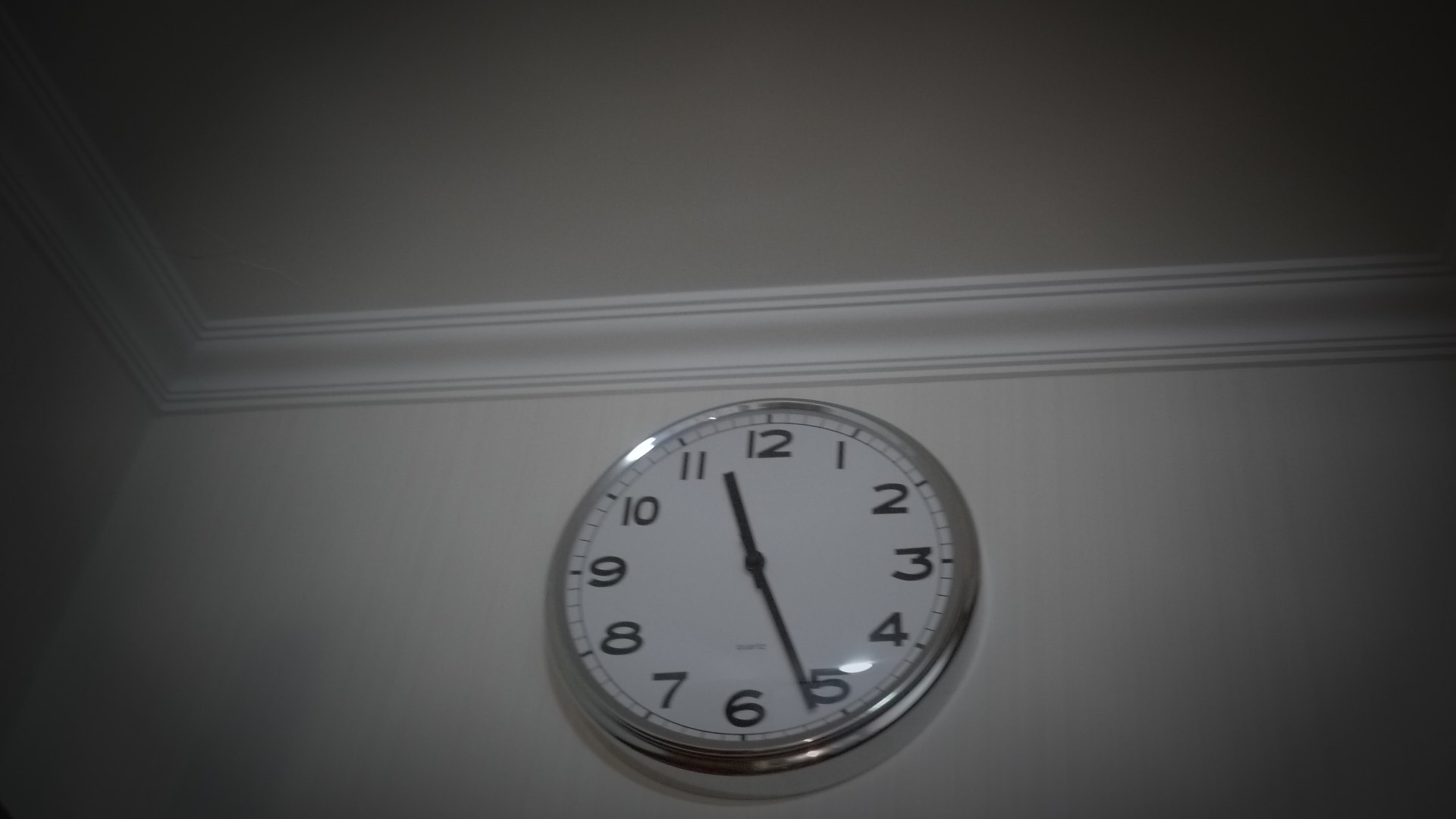This color photograph captures the corner of a residential room, showcasing the intersection of two white walls, with just a sliver of the left wall visible. Prominently featured is a chrome-rimmed, white-faced analog clock with black numbers from 1 to 12. The clock's hands indicate the time as 11:27. Mounted high on the wall, just below the white crown molding, the clock appears slightly illuminated, likely due to a light source shining on it, creating a noticeable glare and giving it a shiny appearance. The image has a vignette effect, with darker edges framing the scene, adding depth and focus to the illuminated clock.